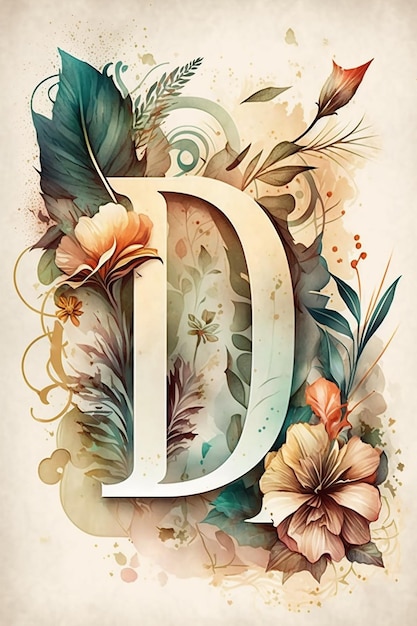The image, likely the front of a greeting card or stationery, features a large, white, intricately designed letter "D" at its center. This "D" is surrounded by a vibrant, artistic arrangement of pink and peach flowers, both bloomed and unbloomed, interspersed with teal green leaves and looping vines. At the bottom right and left sides, larger blossoms with delicate petals extend outward, their centers light and detailed. Smaller red and yellow flowers add depth to the composition, with red specks and small unopened buds dotting the leafy ensemble. The background is a textured blend of brown and cream tones, adorned with swirling green spiral designs and faint watercolor splashes in peach and green. Behind the picturesque floral arrangement, subtle brown dots and green arches contribute an elegant, layered aesthetic, making the detailed, watercolor-inspired artwork rich and visually captivating.